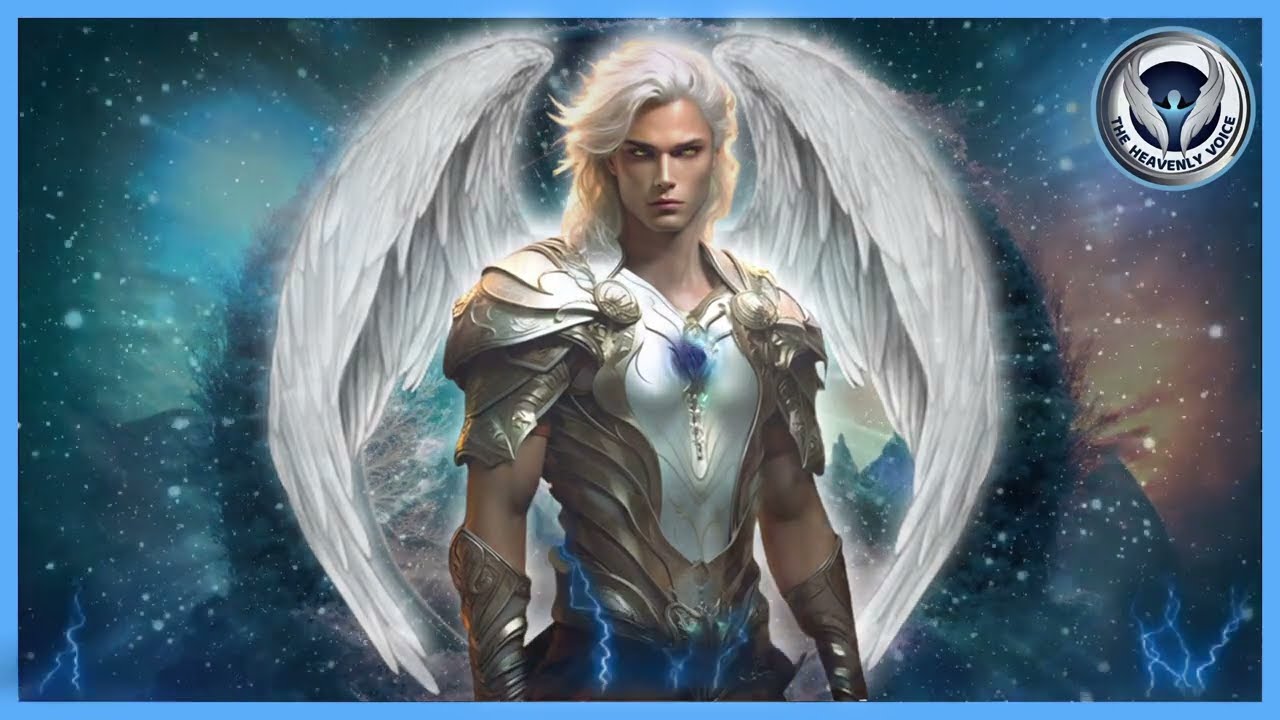The digitally created image features a central figure, a young man with tanned skin, white, flowing hair that glows and sweeps upwards to the left, and supernatural white eyes that are mostly closed. He wears intricate body armor that covers his chest and shoulders, leaving his elbows exposed, with additional armor on his hands. White angel wings extend from the top of his head, arching upward and framing his head before curving downward to his waist. 

The background is a vibrant, abstract design with glowing white dots and distinct color contrasts: blue flashes on the left and orange on the right, with lightning-like strings in the bottom corners. In the upper right corner is a circular emblem featuring wings and a blue center, with the text "The Heavenly Voice" written in black beneath the wings. Surrounding the entire image is a light blue square, enhancing the ethereal and otherworldly atmosphere. The overall sci-fi or fantasy aesthetic suggests influences from video game or anime styles.